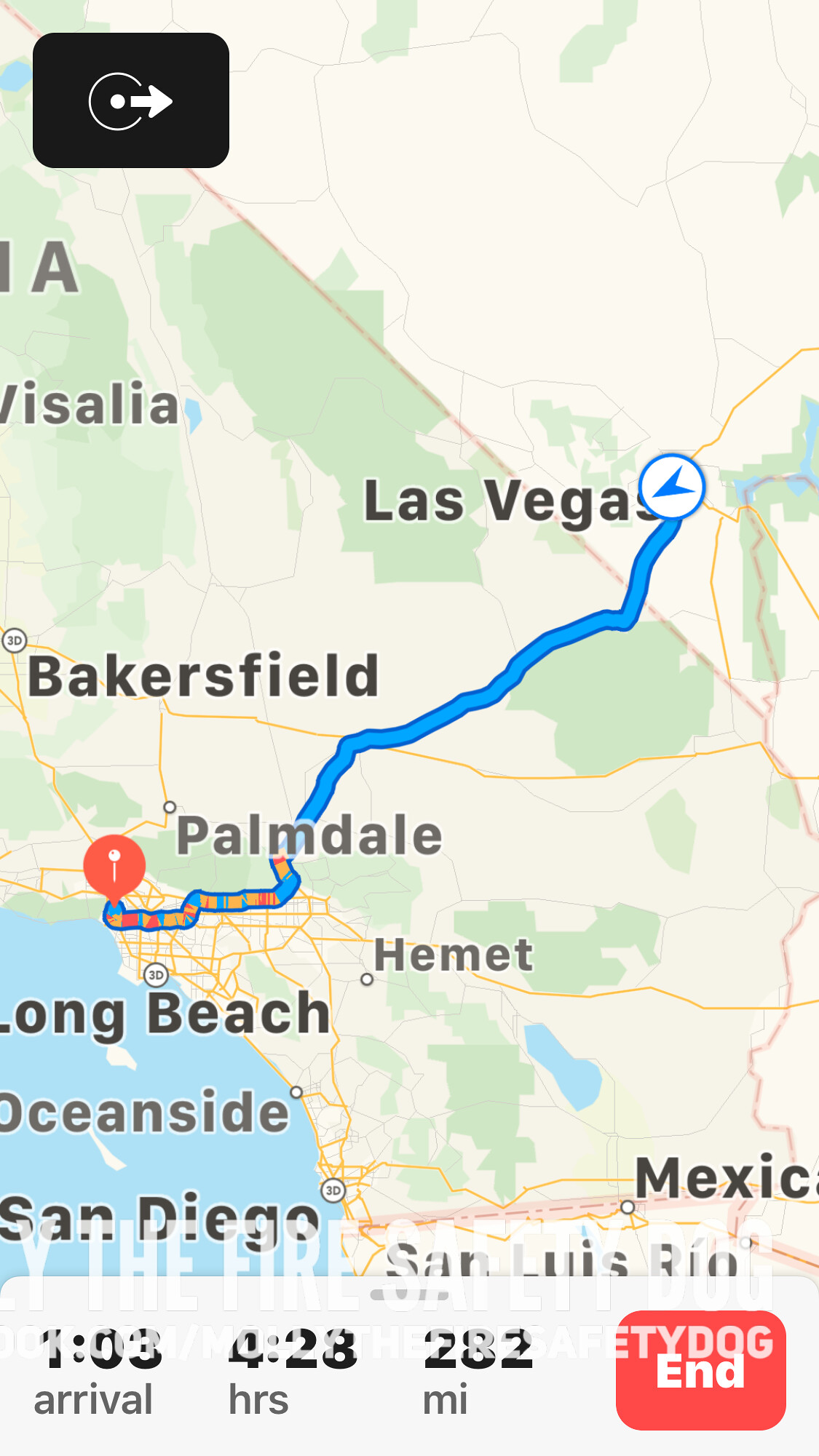This detailed caption comprehensively describes an image captured on a smartphone screen showing a map route from Long Beach to Las Vegas using a map application:

"The image is a rectangular screenshot from a smartphone, displaying a map route from Long Beach to Las Vegas on a navigation app. Imposed on the screenshot is white text, partially cut off on the left, with the readable segment repeating 'the fire safety dog'. This phrase is reiterated multiple times below the incomplete text. At the bottom of the screenshot, there is a gray rectangular banner containing several lines of black text. It reads: '103 arrival for 28 hours, 282 miles'. On the right side of this gray banner, there is a red rectangle with the word 'END' in white.

The map prominently features a blue line tracking the route from the starting point, marked with a pinpoint icon, to the destination, indicated by an arrow icon. In the top left corner of the map, a black rectangle houses a white circle with a right-pointing arrow stemming from a central dot, suggesting a direction or navigation instruction."